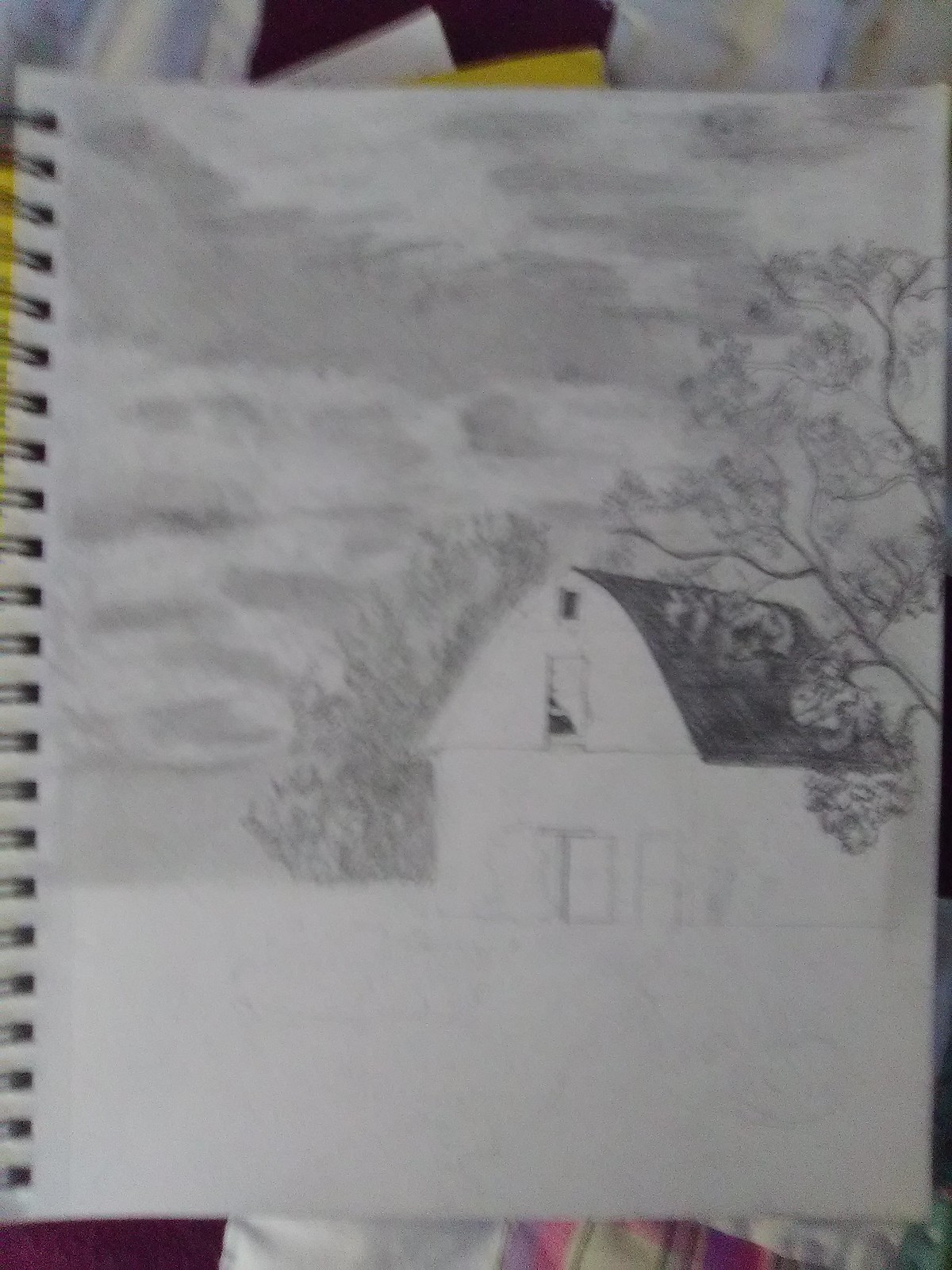In this somewhat blurry image, we see a detailed black-and-white drawing, possibly created on a spiral notebook. The focal point of the drawing is a two-story house or barn, characterized by its white facade and black roof. The sketch suggests a serene rural setting, as evidenced by the depiction of trees to the far right and additional foliage in the background. The sky is rendered in shaded tones of gray and black, adding depth to the scene. Notably, at the top of the image, there appears to be another piece of artwork, distinguished by its black and yellow hues. The bottom portion of the image hints that the drawing might be situated on a tabletop, with indistinct patches of pink and white visible, though their exact nature is unclear. Overall, the artwork showcases a thoughtful composition in shades of gray, white, and black, capturing the essence of a peaceful countryside.